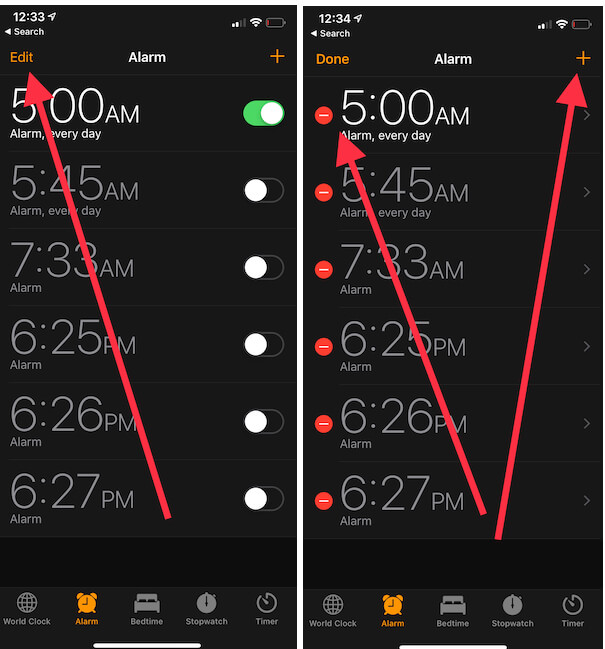The image consists of two side-by-side screenshots from a phone. In the upper left-hand corner of the first column, the time reads 12:33, while in the upper left-hand corner of the second column, it reads 12:34, indicating the screenshots were taken consecutively. 

In the first column, a red arrow points to an "Edit" button at the top, guiding the user on what to press. Below, an alarm set for 5:00 a.m. is toggled on, indicated by a green switch. Beneath this, there are additional alarm times listed: 5:45, 7:33, 6:25, 6:26, and 6:27, all of which have their toggle switches turned off.

In the second column, after pressing the "Edit" button, an orange-highlighted "Done" button replaces "Edit." All listed alarm times are now accompanied by red circles with minus signs, indicating that they can be deleted. Additionally, a red arrow points to an "Add" button, signifying that new alarms can be added.

At the bottom left corner of both screenshots, various icons such as World Clock, Alarm, Bedtime, Stopwatch, and Timer are shown. The "Alarm" icon is highlighted in orange, confirming that the screenshots pertain to the alarm section of the app.